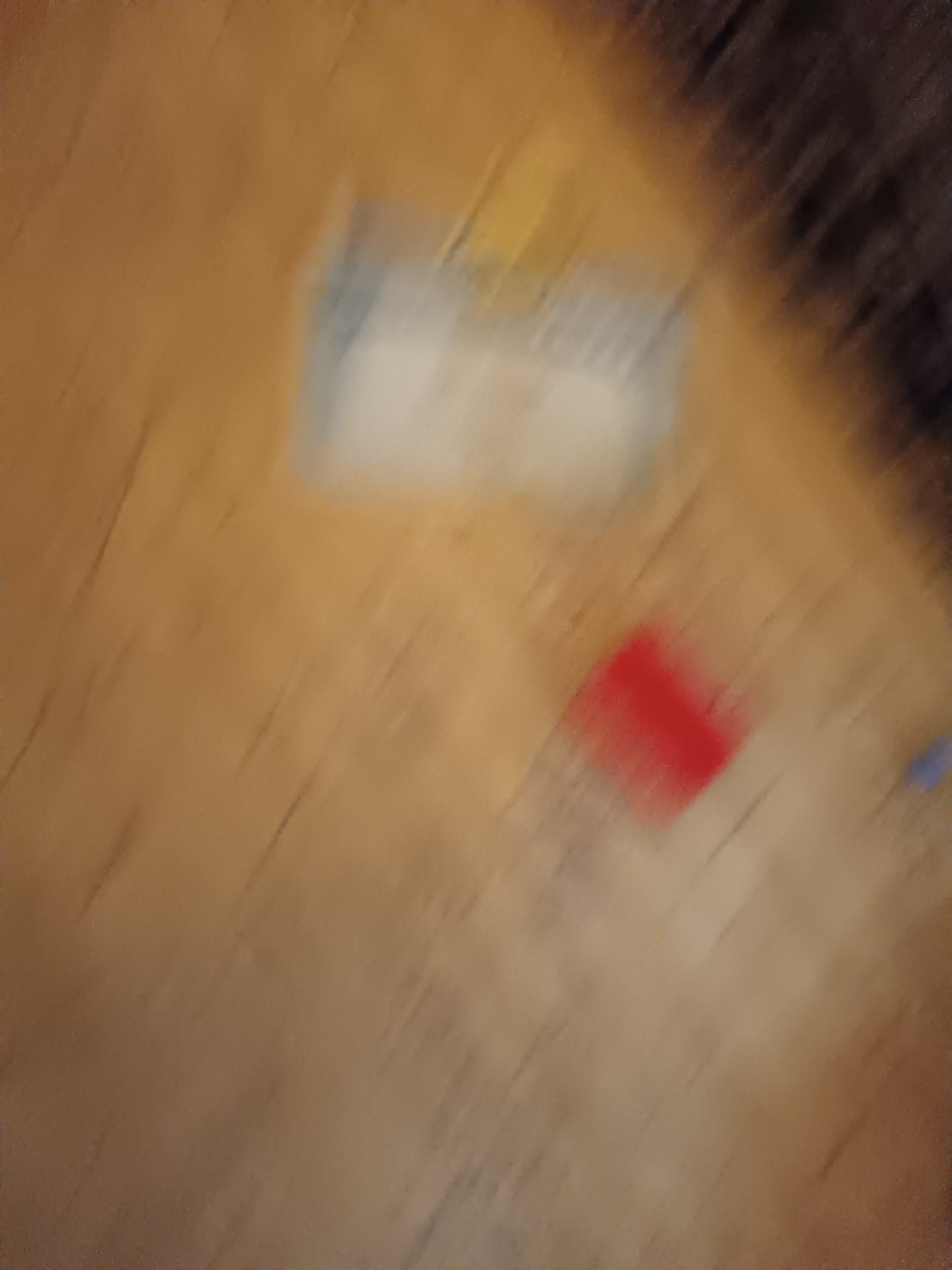This blurred colour photograph depicts two unidentified items laying on what appears to be a wooden table or floor. The background is predominantly a browny, light golden brown hue that is slightly muted at the bottom. Small diagonal lines run upwards from left to right across the image. In the upper right-hand corner, a dark brown triangular shadow extends almost halfway down. Towards the top of the photograph, there's a rectangular white shape with a blue outline, closely resembling a social security card. Below it, there's a small, reddish-orange rectangle positioned almost like a diamond. In the center right edge, a tiny, circular blue object can be seen. The overall blurriness and strong motion lines make it difficult to definitively identify the objects.